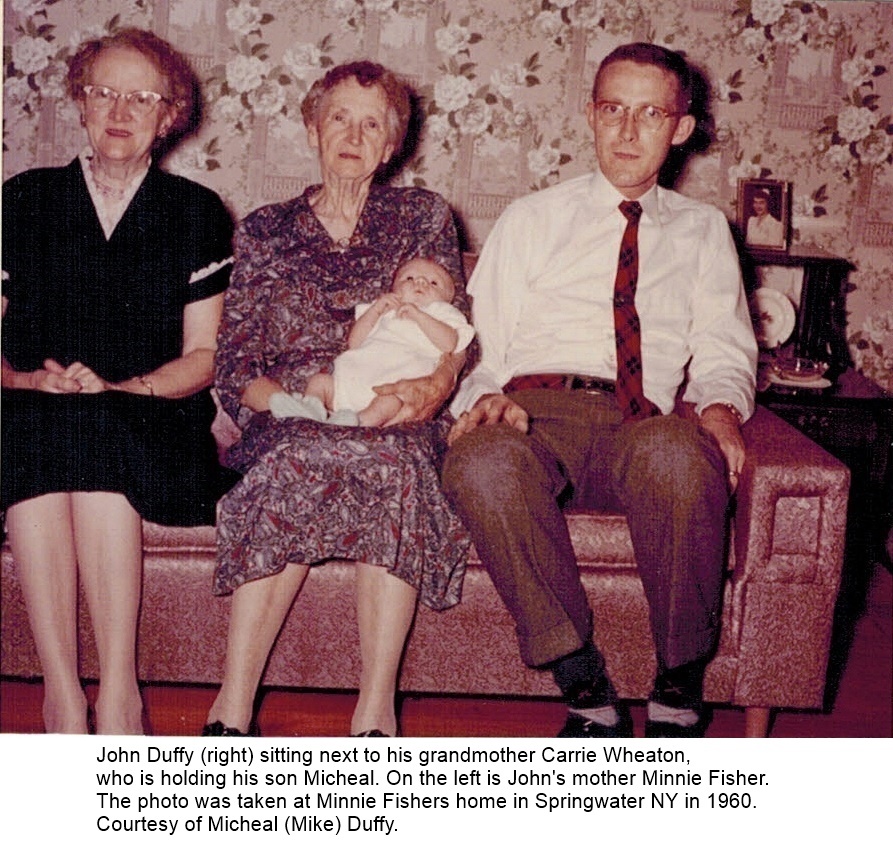This vintage family photograph, taken in 1960, features three adults and a baby seated on a maroon couch against a wall adorned with white floral-patterned wallpaper at Minnie Fisher's home in Springwater, New York. On the left, Minnie Fisher, an older woman wearing a black dress with a white lacy collar and horn-rimmed glasses, sits with a dignified air. Beside her, in the center, is Carrie Wheaton, dressed in a busy, floral print dress, holding the infant Michael Duffy. John Duffy Wright sits on the right, dressed in a white shirt with a skinny red tie, brown slacks, and argyle socks. The red carpeting adds warmth to the cozy scene. A small side table with various items, including a photo frame, stands behind John, adding to the homely feel. The image is accompanied by a caption: "John Duffy Wright, sitting next to his grandmother Carrie Wheaton, who is holding his son Michael. On the left is John's mother, Minnie Fisher. The photo was taken at Minnie Fisher's home in Springwater, New York, in 1960, courtesy of Michael (Mike) Duffy."